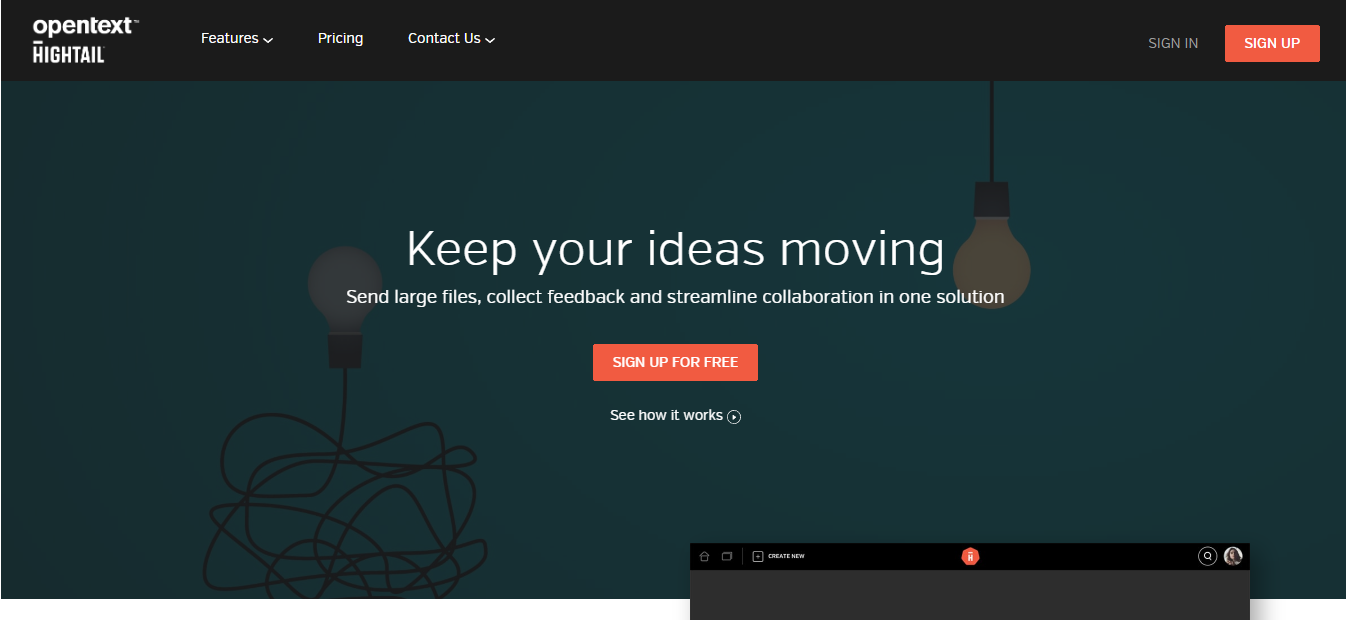### Web Page Description

The webpage features a sleek, modern design with a black bezel running along the top. On the left side of this bezel, the bold, white text reads "OPENTEXT" followed by "HIGHTAIL." Adjacent to these are several navigation tabs including "FEATURES" with a drop-down arrow, "PRICING," and "CONTACT US" also accompanied by a drop-down arrow.

The bezel also contains two rectangular buttons: one black with "SIGN IN" in white text, and another orange with "SIGN IN" in bold white text. Centered prominently on the page, in bold white letters, is the tagline "KEEP YOUR IDEAS MOVING." Below this, in thinner white text, is the description: "SEND LARGE FILES, COLLECT FEEDBACK AND STREAMLINE COLLABORATION IN ONE SOLUTION."

Adding to the visual interest, there is an illustrated light bulb with a black wire on the left-hand side and another light bulb hanging down from the bezel on the top right. An orange button with "SIGN UP FOR FREE" in white text is centrally placed below the main text.

Further down, a section reads "SEE IT" and "SEE HOW IT WORKS" in a mix of bold and thin white text, accompanied by a white circle with a dot in its center. At the bottom of the page, surrounded by a black bezel, is a small rectangular section featuring symbols such as "DELETE," "TWO WINDOWS," and "ANOTHER WINDOW."

Additionally, there is an illustrated hexagon with an orange center and a white object within. Nearby, in a circle, is a white hourglass icon. Finally, a profile picture depicting a light-skinned person with brown hair is displayed above a dark gray rectangle, completing the detailed and visually appealing layout of the webpage.